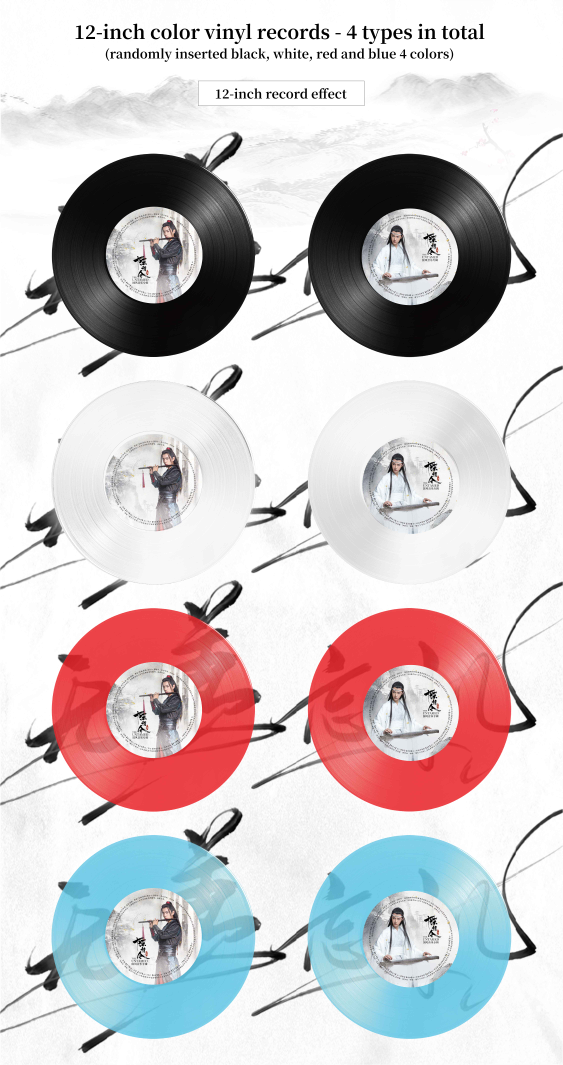The image showcases a collection of eight 12-inch vinyl records, each neatly arranged in four vertical rows. At the top, a line of text in small black print reads, "12-inch color vinyl records - four types in total, randomly inserted: black, white, red, and blue." Directly below this, another line states, "12-inch record effects." Each row contains two records side by side. The first row features two black records, followed by the second row with two white records. The third row displays two red records, and the bottom row contains two teal blue records. All the records share identical labels that feature Chinese characters and caricatures, including a figure blowing a flute and another playing a stringed instrument with long, braided hair. The setting includes a backdrop of a Chinese caricature. Despite their vibrant colors, there is no indication that these vinyl records contain any recorded music.